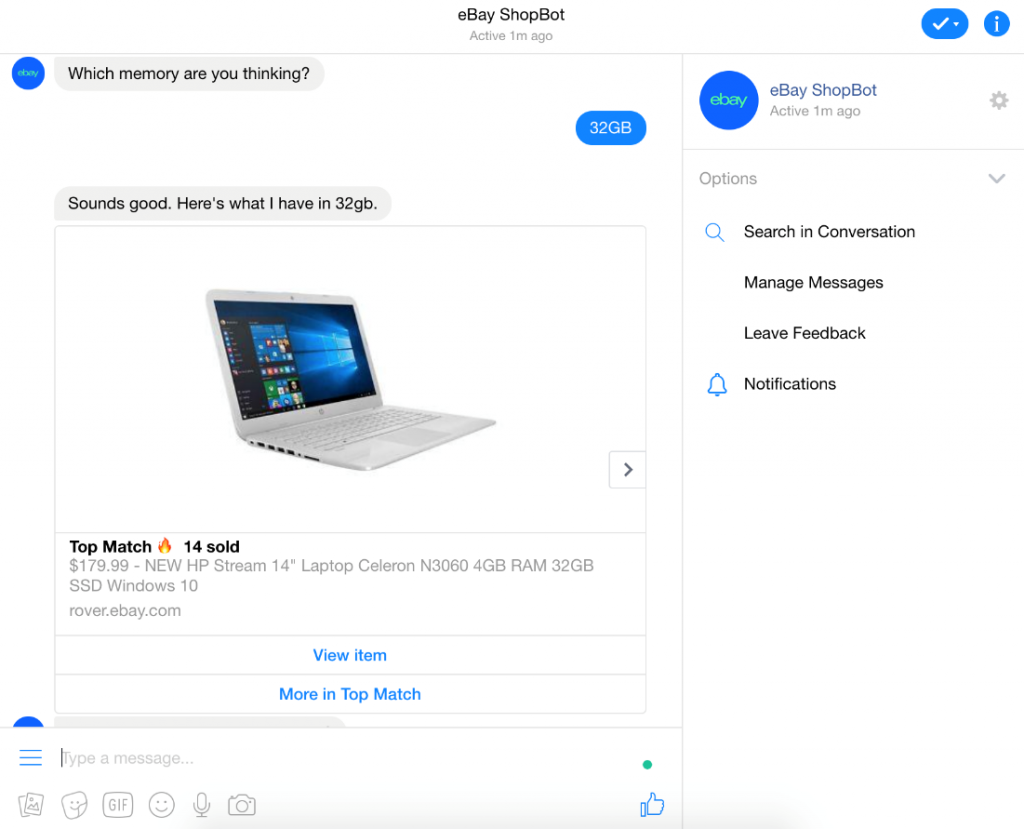**Detailed Caption:**

The image features a clean, white background with various design elements and text associated with an eBay interface. Centered at the top is the eBay logo in black, with a capital "B." Below this, the words "Shop" with a capital "S" and "Bot" with a capital "B" are displayed. Just underneath, also in gray, it reads "active five minutes ago."

To the right of this text, there is a blue oval icon containing a white check mark and a white downward-pointing triangle. Below this, a blue circle encloses a white "i."

Traversing the screen horizontally, there's a thin gray line. Following this line downward, another blue circle appears, this time with "eBay" written inside in green.

Further down, a conversation is depicted. A gray oval contains black text that asks, "Which memory are you thinking?" In response, another blue oval contains white text reading "32 GB." Another reply follows in a gray oval, with black text stating, "Sounds good. Here's what I have in 32 GB."

Visually outlined below the conversation is a gray laptop image. Directly underneath the laptop in black text, it reads "Top match," accompanied by a stylized fire symbol in yellow, orange, and red. Below this, more gray text lists the price and details: "$179.99 - NEW HP Stream 14-inch Laptop, Celeron N3060, 4GB RAM, 32GB SSD, Windows 10." There’s a blue "View Item" button, followed by another blue button labeled "Move" and "Top match."

On the far right, towards the bottom of the image, text in black reads "eBay Shop Bot active one minute ago," followed by various options: "Search and Conversations," "Manage Messages," "Leave Feedback," and "Notifications." Additionally, there is an icon of a blue bell beside the word "Notifications" in black text.